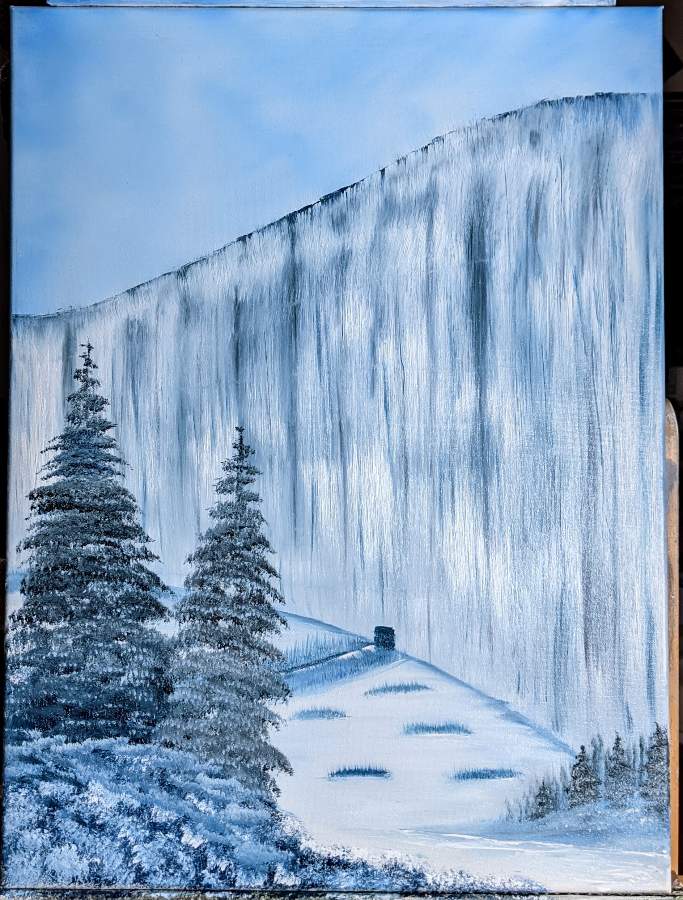This vertical rectangular painting, primarily composed in tones of white and blue, evokes the chilling essence of winter. Dominating the scene is a massive, towering wall of ice or a very white cliffside extending across the middle background. At its base, patches of snow, intermixed with spots of melted ground, reveal underlying grass. To the lower right, clusters of small bushes emerge from the snowy landscape, while the lower left is notable for snow-dusted grass and an embankment.

In the foreground, two imposing evergreen trees, heavily laden with snow, stand prominently on the left, contrasting with smaller pine trees scattered along a lower hill to the right. A tiny black structure, resembling an entrance or a hole, is discernible at the base of the colossal ice wall, reminiscent of an entryway akin to the Night's Watch base from Game of Thrones.

The sky above is a crisp blue, adorned with high, wispy white clouds, further enhancing the painting's cold and serene atmosphere. Earth tones and snow-covered patches interspersed throughout the scene emphasize the winter setting’s stark and beautiful desolation.